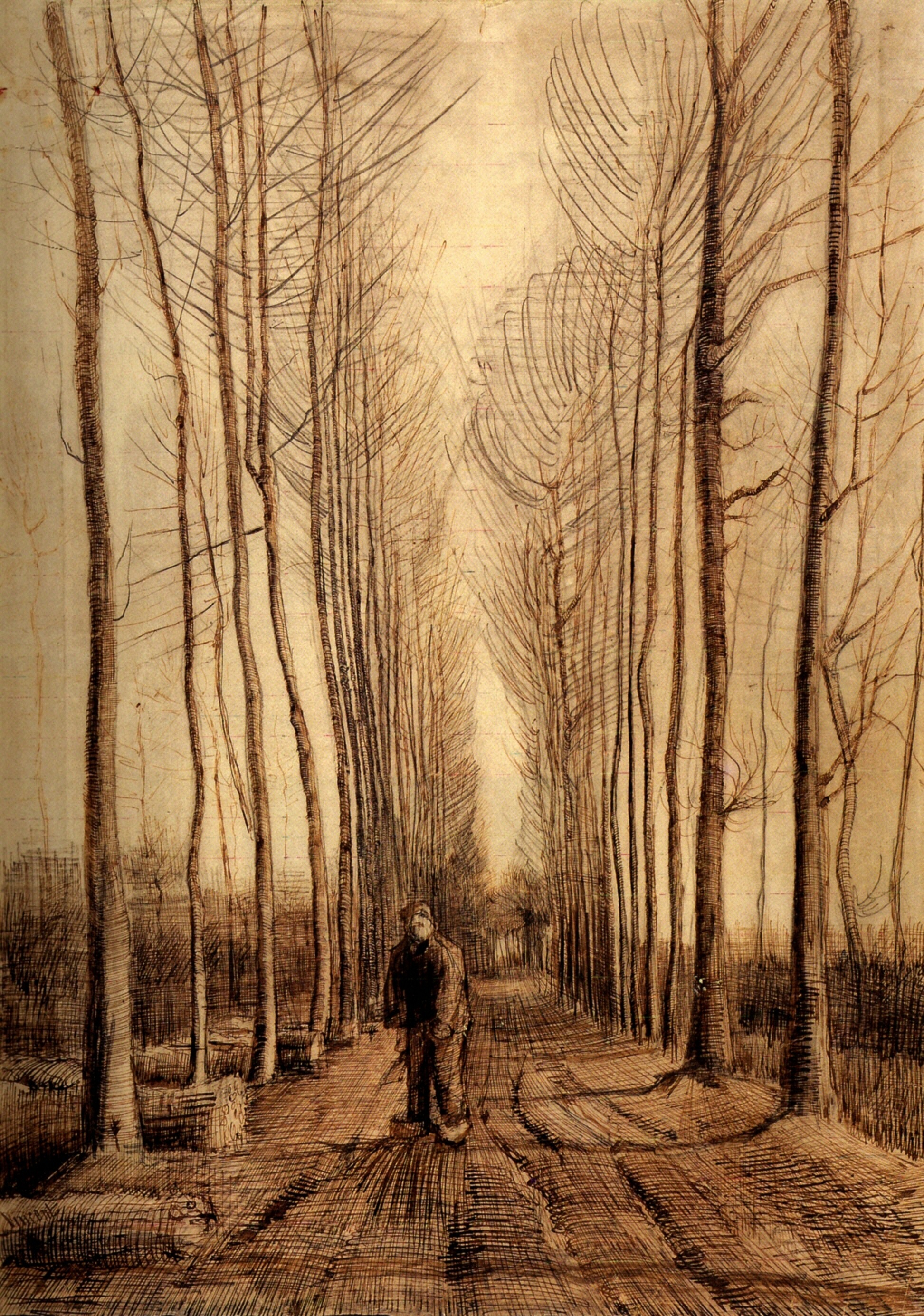The image, possibly a pencil drawing or painting by Vincent van Gogh titled "Avenue of Poplars," showcases an intriguing play of light and perspective. Central to the composition is a solitary man standing on a dirt road, wearing a coat, pants, and a hat, though his features remain indistinct. The road stretches into the distance, creating a vanishing point in the middle of the picture.

On either side of the road are tall, skeletal poplar trees, devoid of leaves and characterized by their thin trunks and sparse, wispy branches. These trees extend in a uniform line, further emphasizing the road's perspective.

The left side of the road features several ambiguous objects that appear to be either felled trees, tree stumps, or bales of hay. They are large and positioned in the gutter or ditch area. To the right of the road lies an open, possibly fallow, farm field, contributing to the scene's barren and desolate atmosphere.

The background is an ecru or cream shade, suggestive of a bright, sunny afternoon. The color scheme is minimal, dominated by shades of white and brown with dark brown shadows and a few touches of orange and black pencil, which create a distinctive, serene mood. Perhaps birch trees, though suggested to be poplars, add to the scene's rustic and primitive aesthetic.